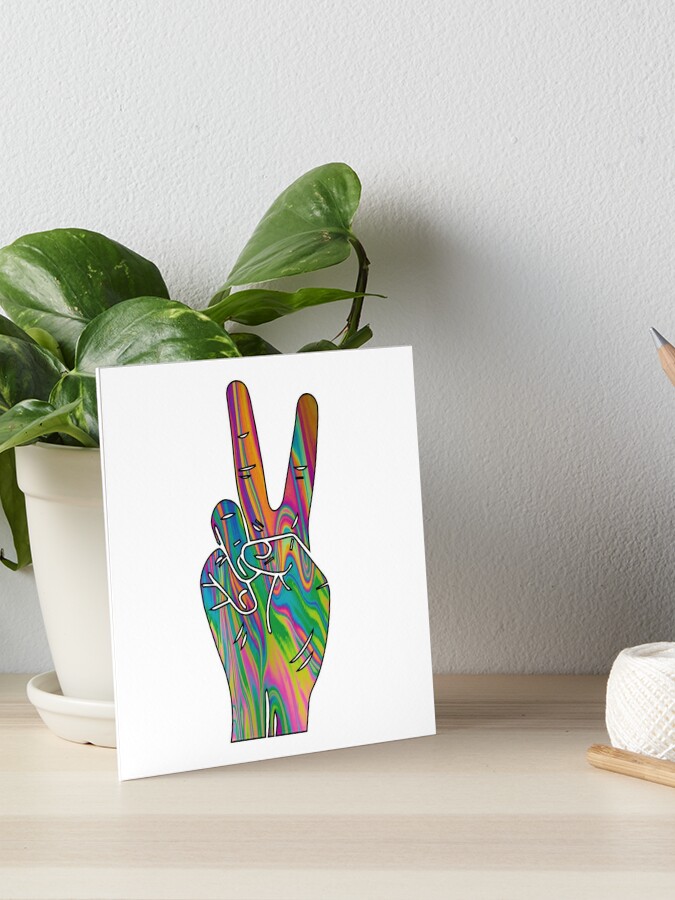This photograph captures a vibrant scene where a small, vertically aligned artwork is propped up against a lush green pothos plant in a white pot. The artwork, a stylized print on white paper, features a right hand making the peace sign with its fingers filled with swirling, psychedelic designs in neon colors including greens, pinks, yellows, oranges, and blues. The background is a textured white wall, while the items rest on a light ivory-colored wooden surface. To the right of the artwork, a white spool of twine is visible, and just above it, the point of a pencil with its lead and brown wood casing is peeking out. The photorealistic setting of the image highlights the contrasting artistic depiction of the hand.